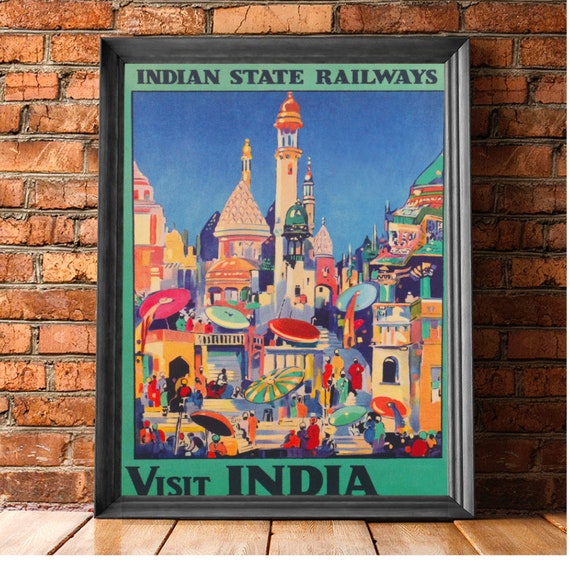This is a photograph of a vintage poster promoting the Indian State Railways with an invitation to "Visit India." The poster rests on a wooden floor, angled against a reddish-brown brick wall. It is framed in a sleek, matte black frame that adds a touch of sophistication to its presentation. The upper edge of the poster features the words "Indian State Railways" in black, prominently displayed on a green background that forms a border around the vibrant scene depicted within.

The central image of the poster bursts with color, showcasing a bustling, idyllic cityscape under a clear blue sky. Rich hues of orange, green, yellow, and red dominate the scene, creating a visually striking tableau. Arrayed across the scene are multiple buildings intricately layered, each adorned in bright, eye-catching colors. A striking feature of the artwork is a tall, slender white tower situated in the middle, capped with an orange bell-shaped top. Flanking this tower are smaller structures capped with green and gold-tinted bell-shaped roofs, respectively.

The bottom of the poster boldly proclaims "Visit India" in black, in all capital letters, inviting viewers to explore the vibrant and culturally rich landscape depicted. The scene also includes numerous people and colorful umbrellas, adding to the dynamic and lively atmosphere of this picturesque Indian city.